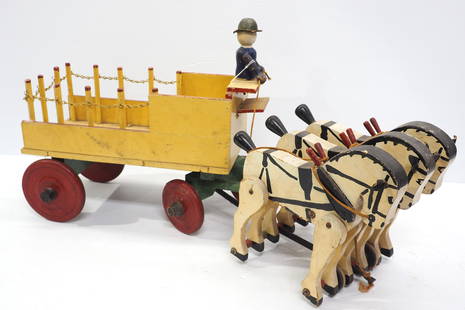The image displays a vintage wooden toy set featuring a bright yellow, gold-hued carriage with red rear wheels and slightly smaller front wheels, connected by green axles. The carriage is embellished with a delicate rope railing at the back, resembling matchsticks, and is being pulled by three identical toy horses arranged side-by-side. These horses are crafted from light brown wood with dark brown manes, tails, and hooves, and are adorned with black saddles and reins. Seated prominently at the front of the carriage is a small toy figure resembling a soldier, distinguished by its blue attire and black hat, serving as the driver. The entire scene is set against a white surface, capturing the intricate details and whimsical charm of this quaint wooden toy ensemble.